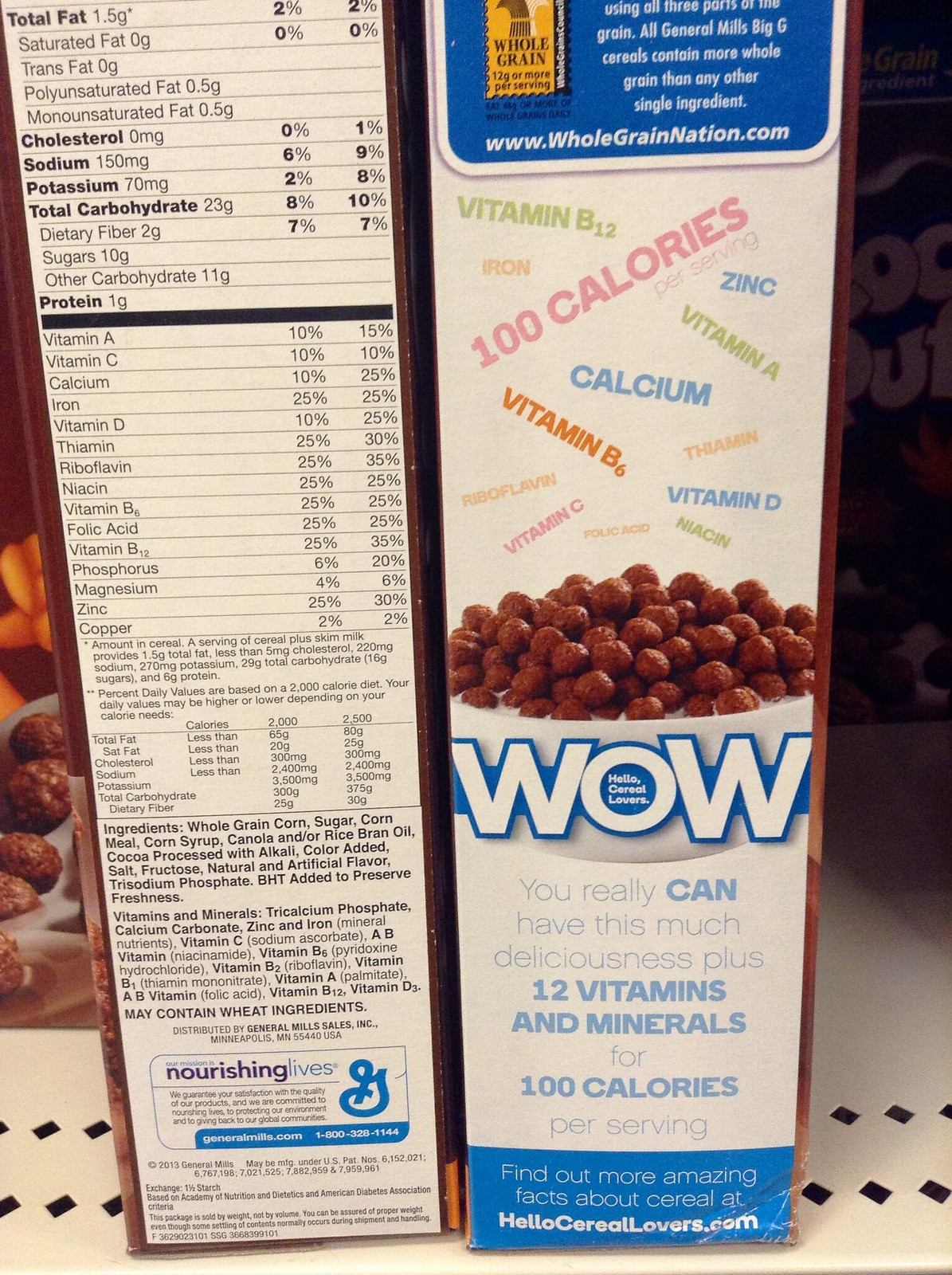This image captures a close-up photograph of two cereal boxes placed side by side on a white metal shelf, vividly illuminated by bright fluorescent lighting. The box on the left is tilted, revealing its side view which displays the detailed Nutritional Facts in black text on a white background. This nutritional information prominently lists values for saturated fat, total fat, cholesterol, sodium, vitamin A, vitamin C, potassium, and includes an ingredient list toward the bottom. The box appears to be for a major type of chocolate puff cereal.

The cereal box on the right presents another side and showcases various marketing advertisements. At the top, a statement proudly emphasizes that the cereal is made from whole grains, alongside a link to the website www.wholegrainnation.com where additional nutritional information can be found. Below this, colorful claims about the vitamins and minerals—such as vitamin B12 (green), iron (light orange), 100 calories (pink), calcium (blue), and vitamin B6—are prominently displayed. A vivid graphic of the cereal itself, which resembles round rice or corn-based puffs, is shown in a bowl of milk. Accompanying this image, bright white text with a blue outline shouts "WOW," followed by an enthusiastic message to cereal lovers about enjoying this delicious cereal with 12 vitamins and minerals for just 100 calories per serving. To the left of the boxes, there is another unidentified food item, while open space stretches to the right, contrasting with the shadows cast on the darker portion of the shelf.